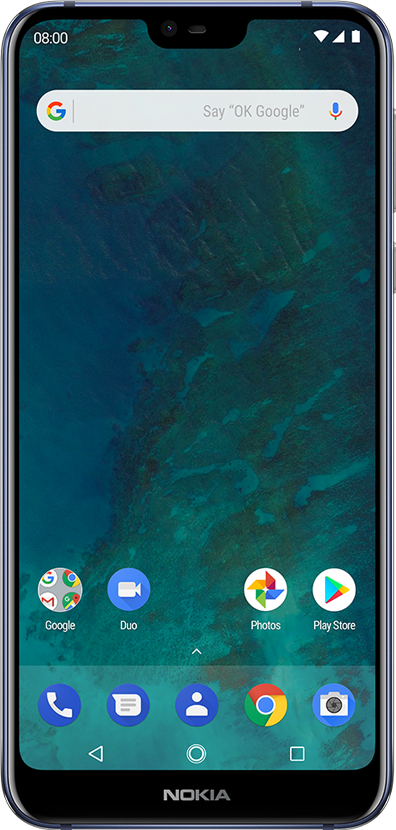A sleek Nokia smartphone is displayed with a vibrant and colorful background reminiscent of ocean waves in various shades of blue. The screen is active, showcasing a detailed user interface. At the top-left corner, the time is displayed as 8 o'clock, while the top-right corner indicates a full Wi-Fi signal, full cellular signal, and a fully charged battery next to a "G" symbol, signifying Google services.

On the home screen, an oval icon prompts the user to "Say 'OK Google'" accompanied by a placeholder text and a microphone symbol, indicating voice command functionality. The screen also features multiple app icons, including Google (G), Chrome, Gmail, and Maps in the top left section.

A prominent blue circle symbolizes a video application, and a pinwheel icon in red, blue, green, and yellow represents Google Photos. The Play Store icon sits in a yellow, red, green, and white color scheme, typical of Google’s branding.

In the bottom segment, a common navigation bar includes a sideways triangle (Back), circle (Home), and square (Recent Apps) from left to right. The Nokia branding is elegantly engraved at the bottom of the phone, reinforcing the iconic Nokia craftsmanship.